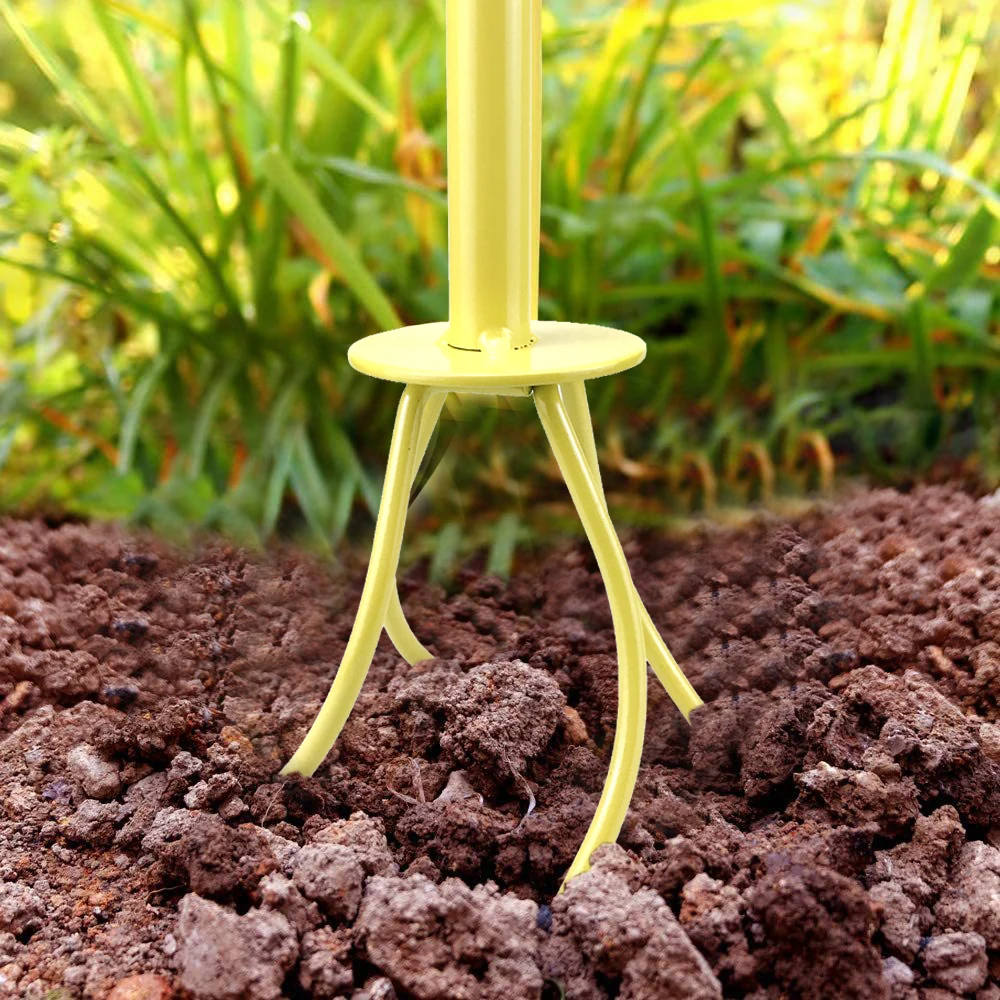The photograph, taken outdoors during the day, captures a bright yellow hand tiller in the foreground, set against a backdrop of lush green vegetation. The tiller, made of sturdy metal, features a prominent yellow pole that extends out of the frame at the top. Attached to this pole is a circular yellow metal plate, from which four spiral-shaped legs or tines extend into the soil below. The dirt is a lumpy, reddish-brown hue, peppered with pebbles and smaller rocks. In the distance, out of focus, are various green plants with broad fronds and grassy foliage, hinting at a garden setting. The tool's design suggests it is used for loosening and aerating the soil, making it more suitable for planting.